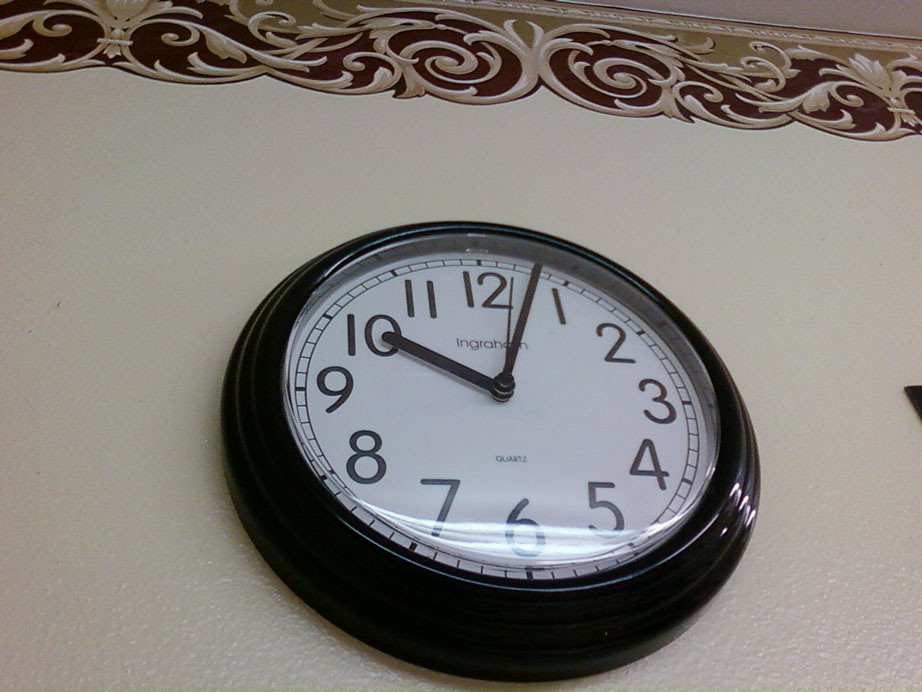This rectangular, landscape-oriented photograph captures a close-up view of a wall-mounted clock. Taken from an upward angle just below the clock, the image reveals its predominantly black exterior casing, contrasting sharply with its pristine white face. Black numerals and matching black dials depict the time as 10:03. Mounted against a white wall, the clock stands as a stark centerpiece. Above the clock, an ornate strip of dark red and gold wallpaper, featuring intricate designs, introduces an element of opulence to the otherwise minimalist setting.